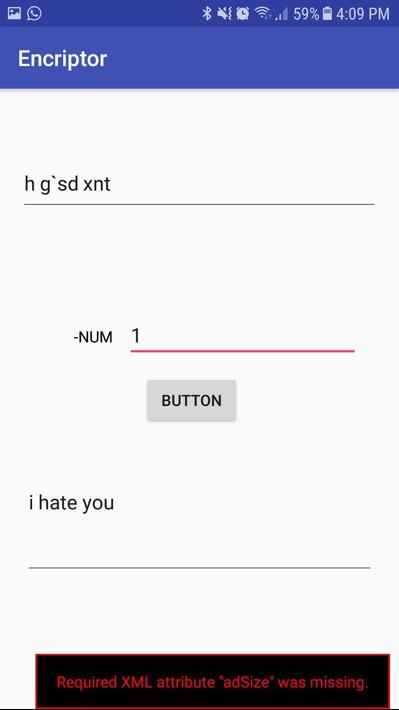The image displays a mobile phone screen with various icons and text. At the top left corner, there is a square icon of an unclear nature, followed by a chat bubble icon containing a phone receiver. The rest of the top section features additional icons on a dark blue background, including a Bluetooth icon with a slash through it, an alarm clock icon, a Wi-Fi signal icon, and a cell phone signal icon. The battery level is indicated as 59% next to a battery icon, and the time displayed in the upper right corner is 4:09 PM.

Below this, a lighter blue background section features the word "Encryptor" in white text. Directly below it, in dark text, is "HG'SDXNT", followed by a horizontal line underneath. The middle portion of the screen shows "−NUMN1" with a red line under the number one, accompanied by a rectangular button labeled "button".

Further down, in dark type, appears the text "I hate you" with another horizontal line below it. At the very bottom of the screen, a black rectangle bordered in red contains a message in red letters: "required XML attribute 'ad size' was missing."